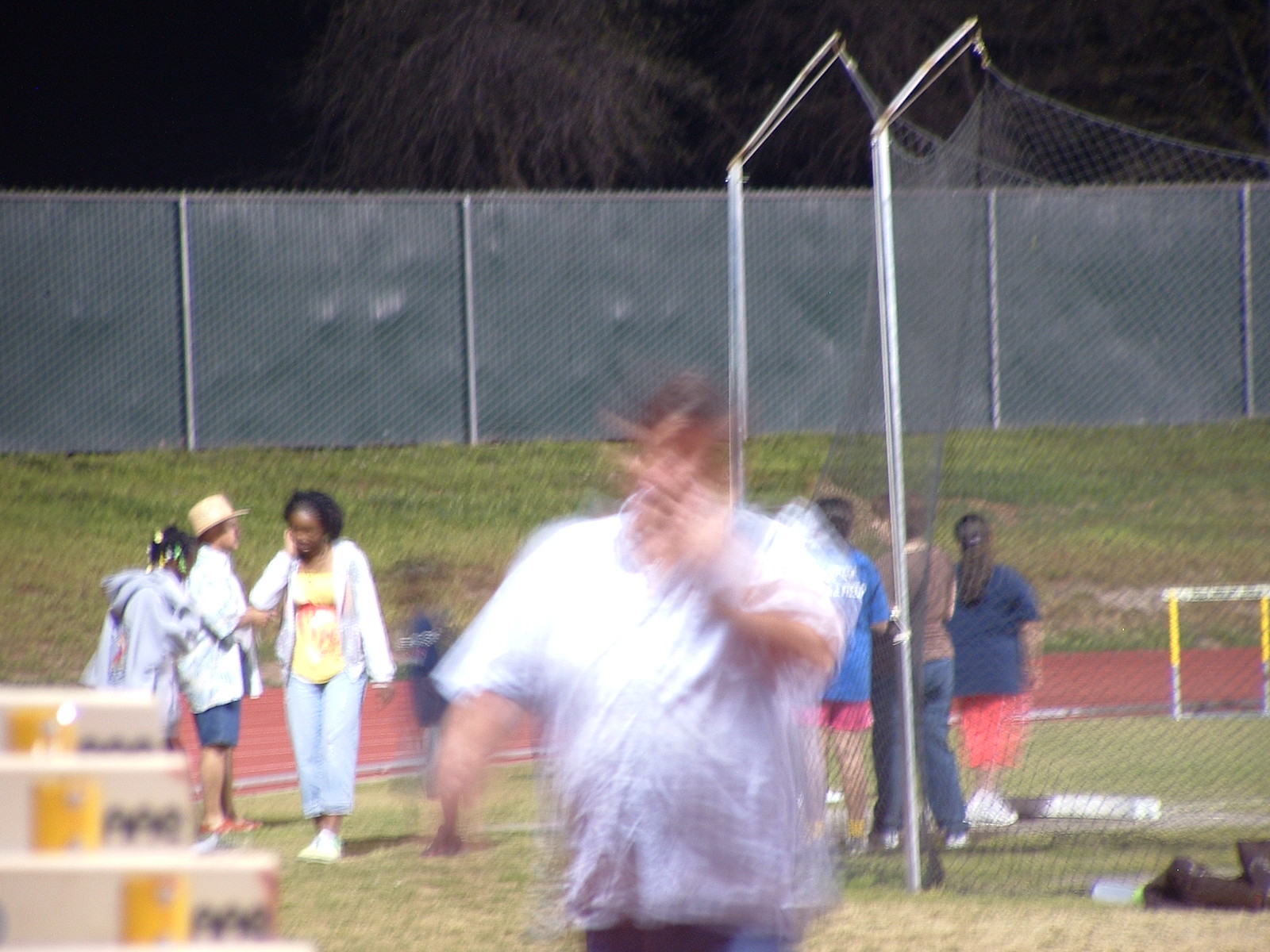In this somewhat blurry image, we see a playing surface that appears to be well-maintained and possibly lawn-mowed. A tall mesh net divides the area, suggesting it could be a sporting ground. Scattered across the scene are individuals dressed in varying athletic attire: some in white, others in blue sporting pink skirts or shorts, and a few on the left-hand side wearing blue shorts. This indicates the presence of two distinct teams. While the exact nature of the sport is unclear due to the absence of identifiable markers like croquet hoops, the setup suggests a form of team-based outdoor activity not easily recognized as typical in the UK. Central to the image is a person in a very white shirt moving forward, though the motion blur lends an unusual quality to their appearance, especially around the hand, giving an impression it has been digitally altered or distorted.